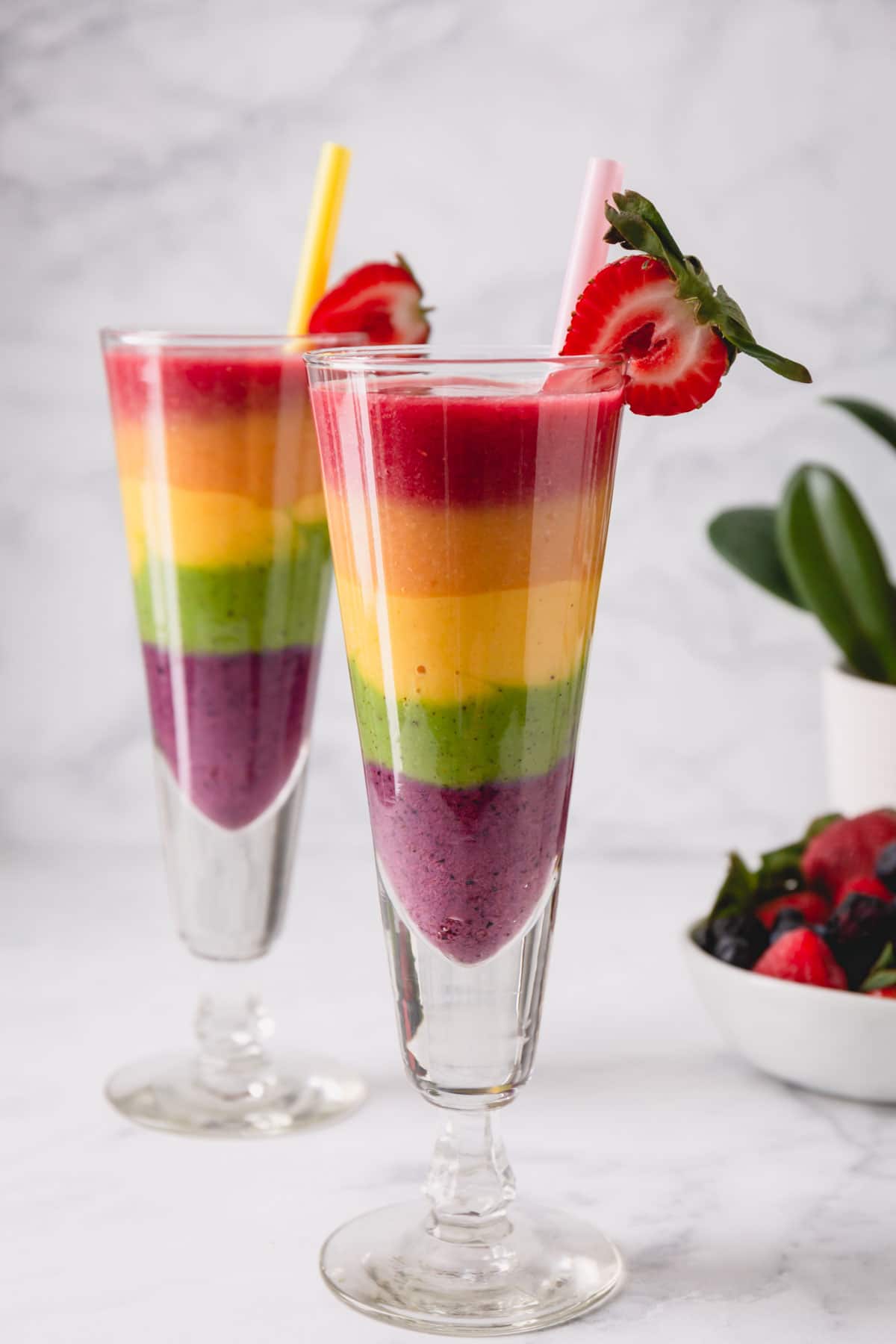The image depicts a beautifully staged, social media-ready scene featuring two elegantly layered smoothie parfaits in slender dessert glasses reminiscent of champagne flutes, each garnished with a strawberry slice and a straw. The parfaits are meticulously arranged with vivid, thick layers of frozen fruit, beginning with a dark purple layer, likely grape, followed by a green layer, possibly kiwi. The next layer is a vibrant yellow, suggesting mango, topped by a bright orange layer, and crowned with a striking red layer, likely strawberry. The parfaits rest on a sleek marble tabletop, accompanied by a small bowl of raspberries and blueberries, and a petite cactus plant, enhancing the overall aesthetic appeal.